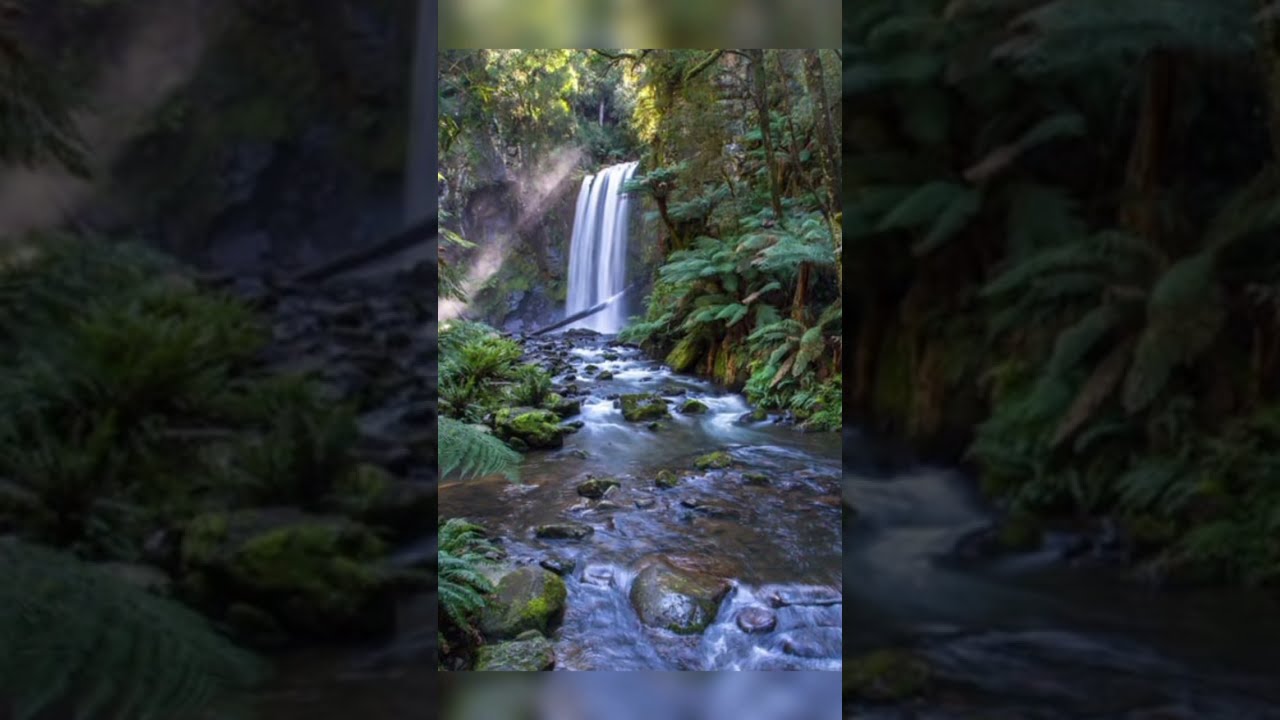This detailed portrait-mode color photograph depicts a serene, lush forest scene centered around a modest yet captivating waterfall. The waterfall, approximately 20 feet high, cascades into a dark, tranquil creek or river, surrounded by a dense array of ferns, bushes, and trees. The scene is largely shaded, with a few beams of sunlight piercing through the thick foliage, adding a touch of brightness to the verdant landscape. In the foreground, large brown and green boulders and rocky outcrops jut out from the river, and the stream flows smoothly towards the viewer.

The photograph is bordered by bands that feature darkened, grayed-out details of the central image, creating an artistic frame that accentuates the vibrant scene within. The trees, characterized by slim brown trunks and green leaves, and ferns are prominently displayed on either side of the stream, adding to the natural richness of the setting. Despite its undeniable beauty, the area does not seem easily accessible nor is it part of a trail, suggesting a hidden gem within a thick, untouched forest. The overall impression is one of tranquil seclusion, further emphasized by the light filtering softly through the tree branches onto the green and black rocks below.